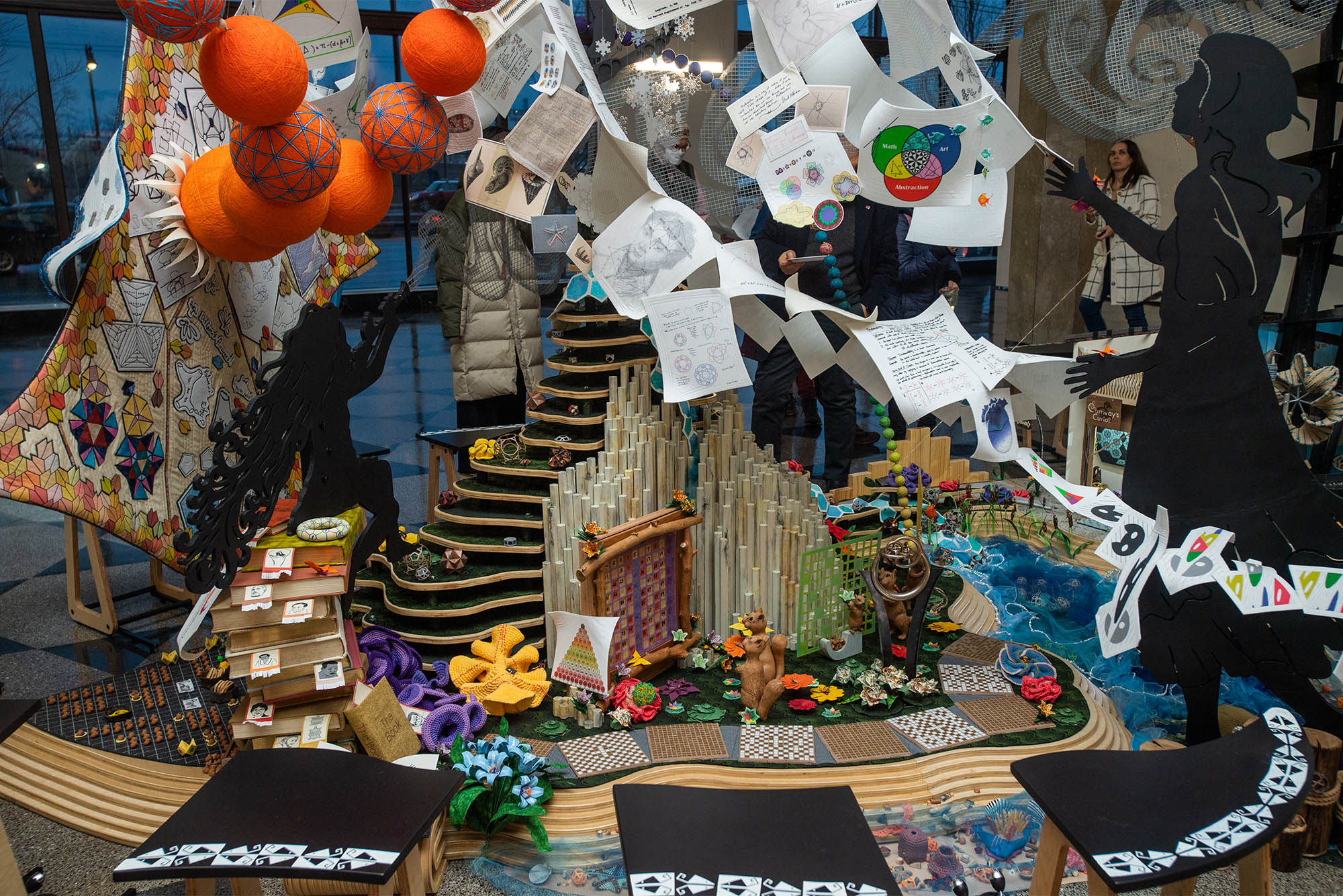This horizontal photograph captures an intricate art installation located inside a spacious building. The art piece is an elaborate assemblage of 3D items meticulously arranged to create a multifaceted visual experience. Prominently featured are papers adorned with various objects, black and white portraits, wheel-like figures, text, and scientific journal graphs, all suspended on ropes. To the right side of the image stands a black silhouetted figure with white lines accentuating her arm and hairline, appearing to hold the ropes.

At the heart of the installation, numerous wooden dowels of varying heights form a mountain-like structure. This central formation includes a vertically-oriented, round rectangular object with a brick-patterned back. In the foreground, small figures and tiles are aligned horizontally.

To the left, the scene includes puzzle pieces and a stack of books. The background reveals a curved, tiered structure with an earthy brown facade, contrasted by its black surroundings. Large, vibrant orange balls are suspended in the upper left corner, hanging in front of a quilt-like material that adds texture to the backdrop. This detailed and dynamic art piece masterfully combines different elements and textures, creating a visually captivating experience.